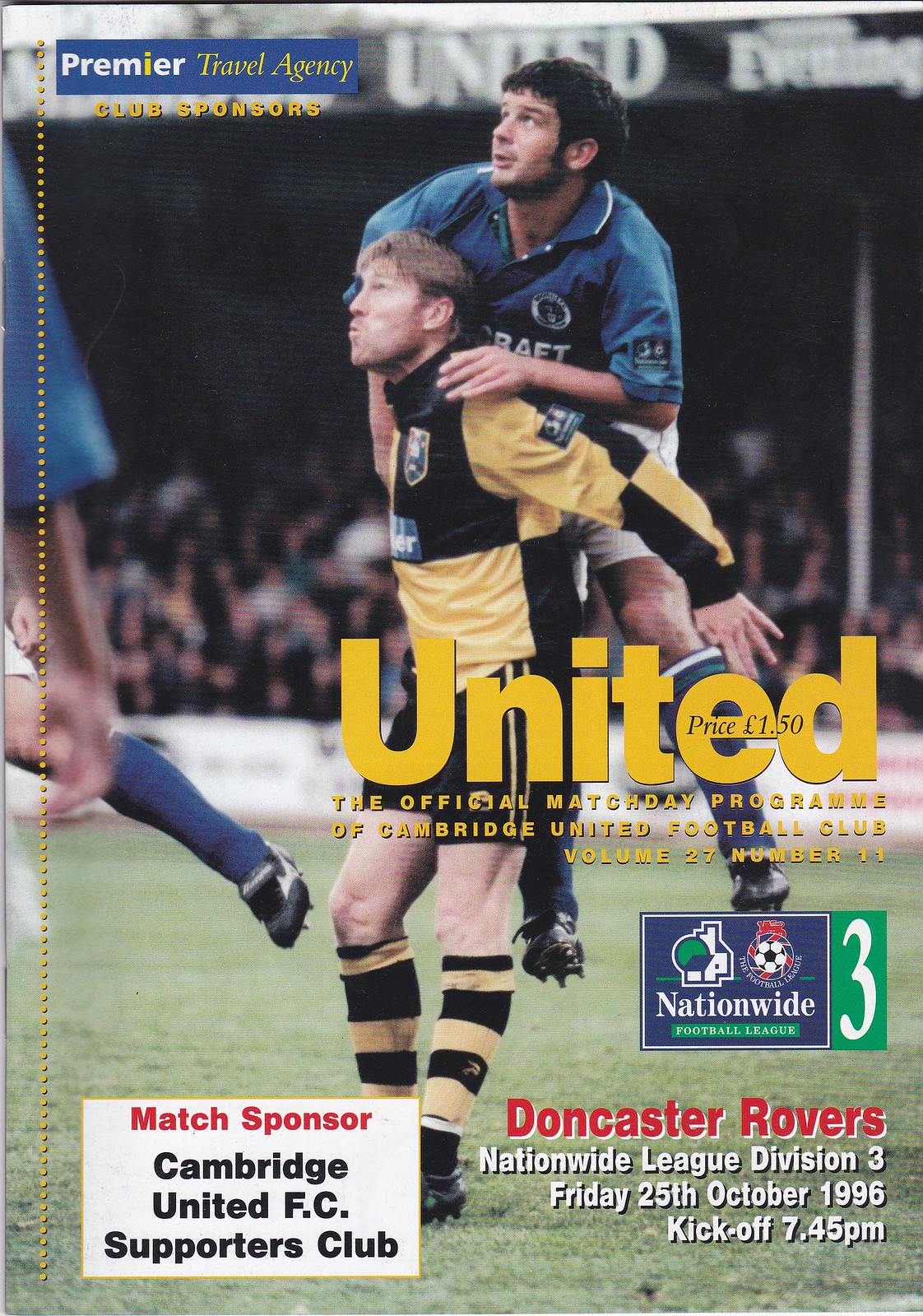This magazine cover features a dynamic image of a soccer match. Central to the scene are two soccer players: one with strawberry blonde hair donning a yellow and black checked long-sleeved jersey and matching striped socks, and another player with brown hair and sideburns, wearing a blue jersey, jumping on his back. They appear to be engaged in the game, possibly looking at an airborne ball, all set on a green grass field with a blurry white barrier and spectators in the background.

Prominently displayed in bold yellow text across the middle of the cover is: "United," followed by "The official match day program of Cambridge United Football Club, Volume 27, Number 11." The top-left corner features a blue rectangle with the text "Premier Travel Agency" and below it in yellow, "Club sponsors." 

In the lower left corner, there is a box stating, "Match sponsor: Cambridge United FC Supporters Club." On the right lower corner, additional details read, "Doncaster Rovers Nationwide League Division III, Friday 25th October 1996, kickoff 7:45 p.m."